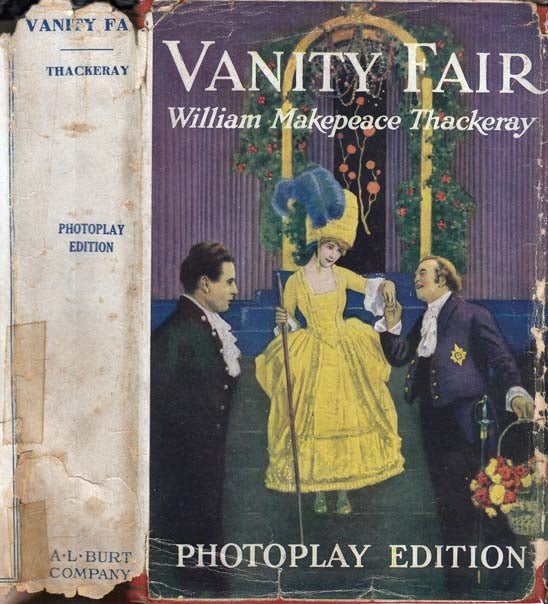The image depicts a worn and partly torn dust jacket of the novel "Vanity Fair" by William Makepeace Thackeray. The dust jacket, showing signs of age with wrinkling and tape repairs, includes both the spine and the front cover. The spine of the dust jacket is white with blue text reading "Vanity Fair" at the top, followed by "Thackeray," "Photo Play Edition" in the middle, and "A. L. Burt Company" at the bottom. The spine also has visible scotch tape repaired areas.

The front cover features an illustration: a woman in a large yellow dress adorned with a matching hat decorated with blue feathers holds a cane in one hand and extends her other hand to a man in a blue suit with a puffy white shirt. This man, who appears to be about to kiss her hand, also holds a basket of red and yellow flowers. To the woman's other side stands another man in a black suit with a puffy shirt, observing the interaction. The background includes an archway draped with vines, flowers, and a purple curtain.

The text on the front cover reads "Vanity Fair" at the top, "William Makepeace Thackeray" below it, and "Photo Play Edition" at the bottom. The entire cover conveys a sense of antiquity and historical aesthetics, characteristic of a much-handled and cherished book.